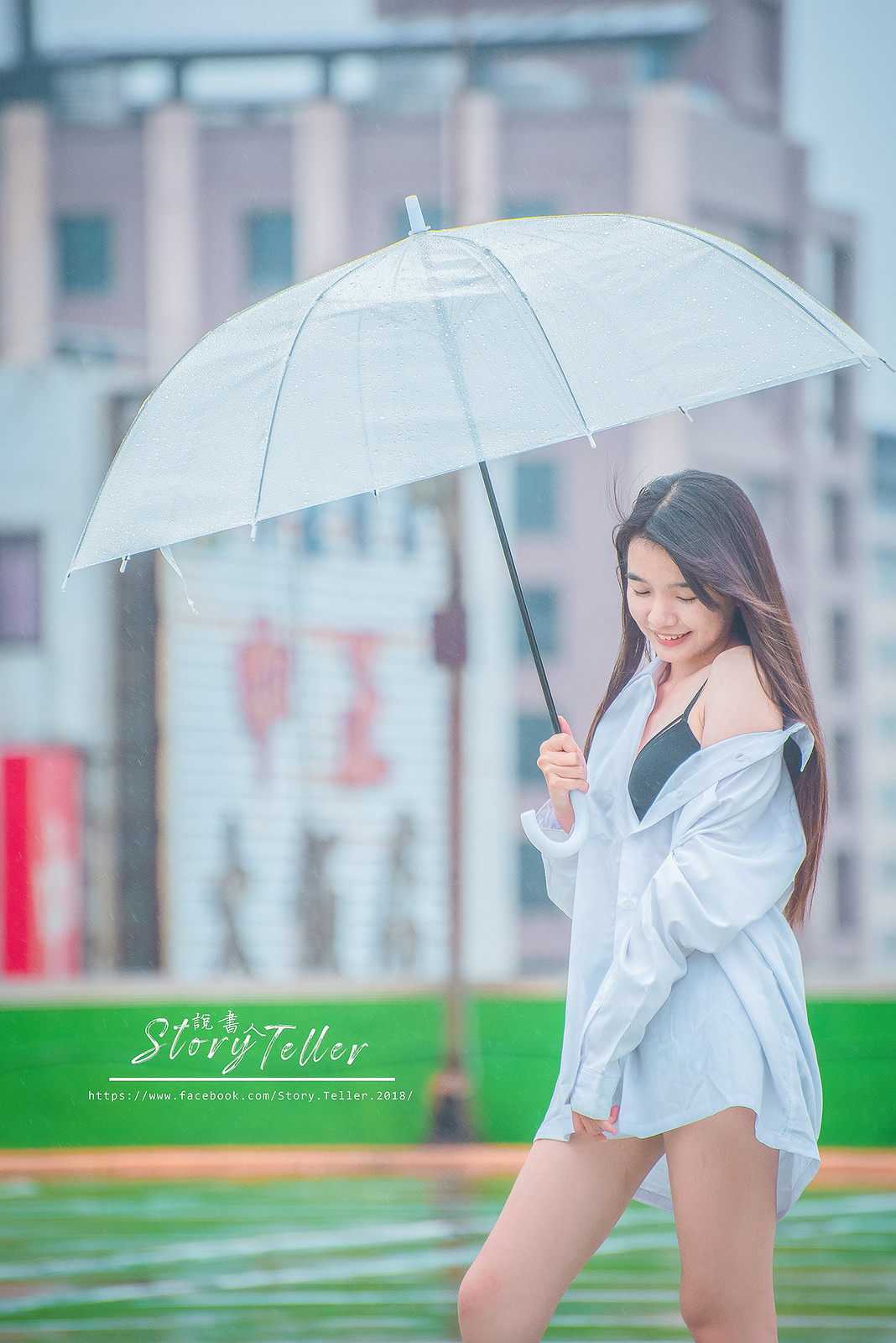The image features a young Asian woman with long, straight brown hair, which extends down her back, covering her ear. She is looking down while holding a semi-transparent gray umbrella with a black handle over her head in her right hand. Her attire consists of an oversized light gray dress shirt that is halfway unbuttoned and slipping off her left shoulder, revealing a black tank top underneath. Her legs appear bare, highlighting her fair skin. The backdrop shows a blurry building with pink and white sections, complementing a field of out-of-focus green grass. In the bottom left corner of the image, the text "Storyteller" is displayed along with a web address, "facebook.com/storyteller.2018". The overall scene suggests an outdoor setting, possibly part of an advertisement or promotional material.